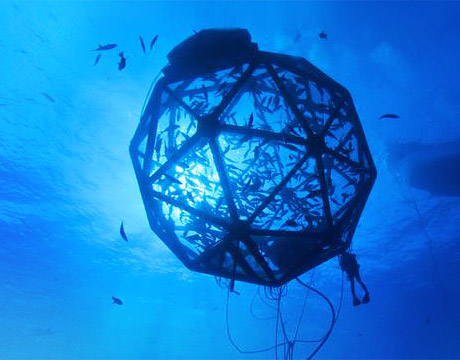This underwater photograph captures an intriguing scene centered on a large, spherical enclosure composed of transparent, triangular panels, resembling a geodesic dome. The structure, deployed in the middle of the ocean, holds a multitude of fish within and around it, suggesting it functions as a fish-catching pod or net. Numerous cables hang from the bottom of the enclosure, extending downwards into the depths of the ocean. In the bottom right corner, a scuba diver, identified by their flippers, hovers near the enclosure, adding a sense of scale and human presence to the scene. To the right of the pod, near the surface, the outline of a boat is faintly visible, connected to the enclosure by a rope. The sun’s rays penetrate the water, creating a stunning glare and illuminating the pod and the marine life within with a gentle, bluish tint.